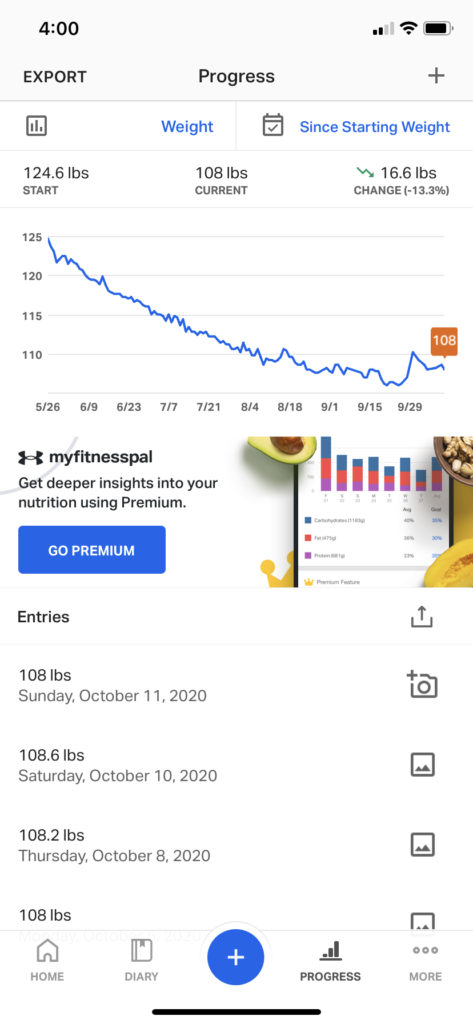This image is a screenshot from a phone displaying a weight tracking app. At the top of the screen, there's a gray header. On the top left, it displays the number "400," and below it, the word "export" is clearly visible. Centrally located in the header is the word "progress." On the top right corner, the phone status indicators show two signal bars, a full Wi-Fi signal, an almost fully charged battery icon, and a plus symbol underneath these indicators. 

Directly beneath the gray header is a thin gray line, followed by a white-bordered section. This section contains fields labeled "Weight" and "Starting Weight." To the right of these labels, there's an area designated for user input. Below this input field, the text indicates "124.6 pounds start" on the left side and "108 pounds current" on the right, with the calculated change of "-16.6 pounds" displayed. The detailed weight change is specified as "-13.4 pounds."

Towards the bottom of the screenshot, there's a graph that charts weight progress over time. The Y-axis on the left side of the graph is marked with numbers ranging from 125 to 110, representing weight in pounds. The X-axis at the bottom of the graph shows dates, with the numbers ranging from 5/26 to 9/29, indicating the time span over which the data was recorded. The image appears somewhat blurred, particularly the fine details, but these are the key elements visible in the screenshot.